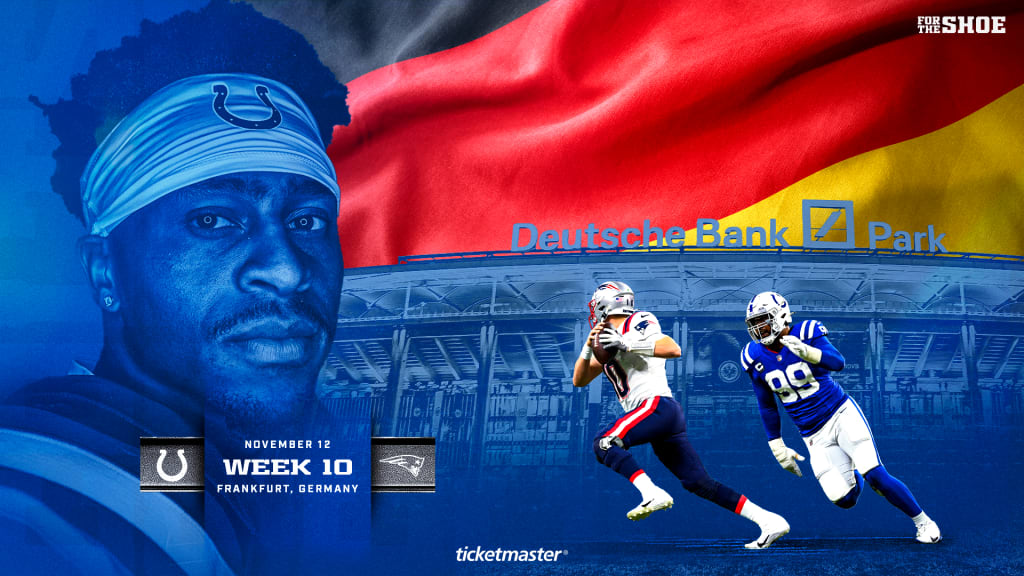The image prominently features a backdrop with the German flag in the upper center-right, displaying dark blue or black at the top, red in the middle, and yellow at the bottom. The scene is set in a stadium filled with blue tones. On the left side, an athlete's face, distinctly a Black man rendered in blue, is visible, wearing a headband and a scarf adorned with a horseshoe logo, reminiscent of football shoulder pads. Prominently displayed on the right are two football players: one in a blue jersey with white pants marked by blue stripes, identifiable as a Colts player wearing number 99, and another in a white jersey with red and blue stripes, representing the Patriots. In the background, the Deutsche Bank Park signage, featuring its logo – a square with a diagonal line – can be seen. Text on the upper right states "For the Shoe" over the German flag. Additionally, the Colts and Patriots logos are visible along with the text “November 12th, Week 10, Frankfurt, Germany." The advertisement for Ticketmaster appears below, completing the vibrant and detailed promotional image.